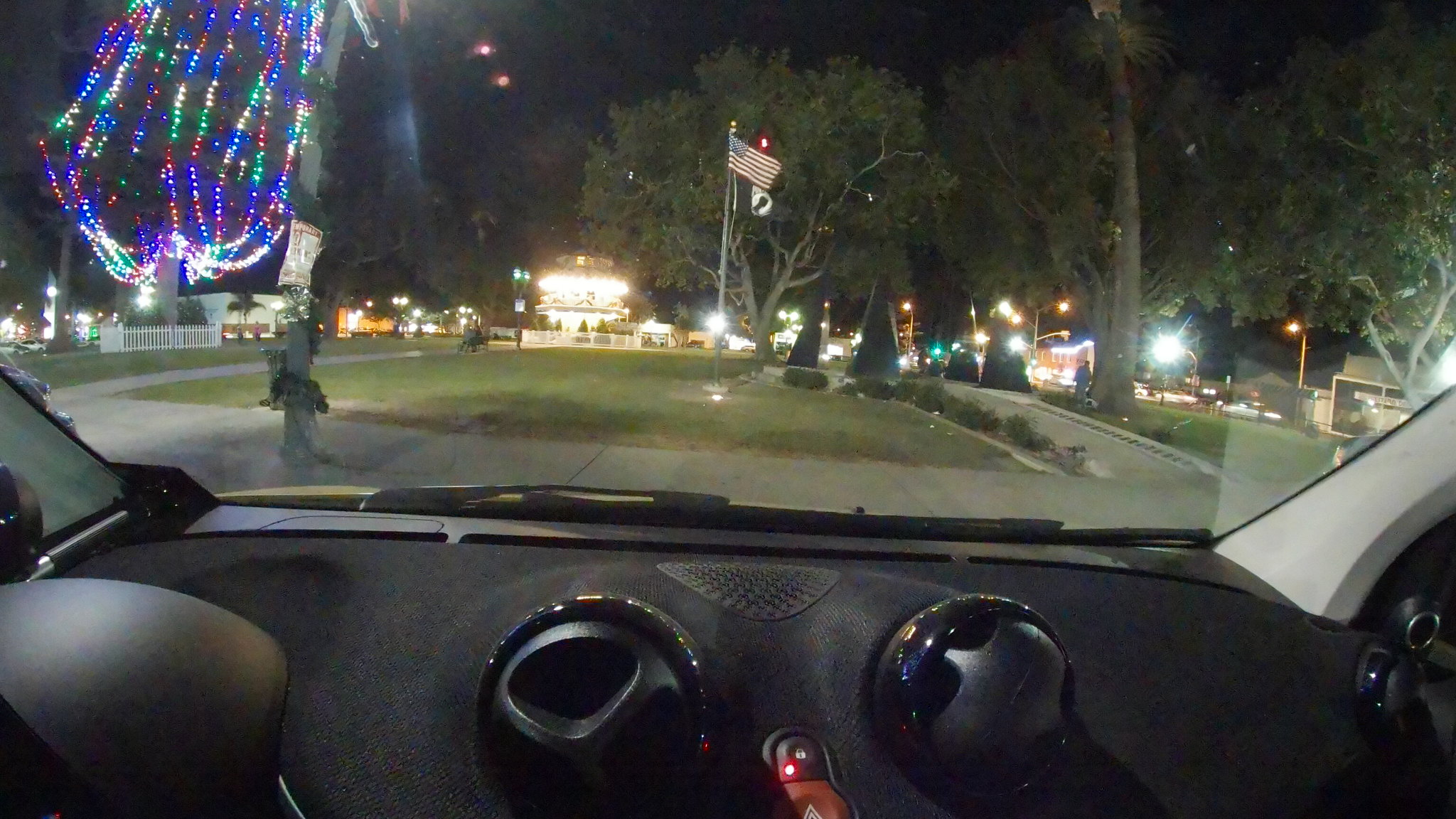This image captures the interior of a vehicle, focusing on its black dashboard. Prominently featured are two circular ventilation vents side by side, situated above a striking red button. Through the windshield, a gray sidewalk stretches horizontally across the foreground, flanked by two vertical sidewalks, one on each side. Nestled between these sidewalks is a patch of green grass adorned with a gray pole, from which the American flag proudly waves.

Further into the background, a tree with dark green leaves stands tall behind the flag, accompanied by two more trees to its right. On the left side, a structure illuminated with blue, yellow, white, and green lights occupies the top left corner, with a white fence beneath it. The sky is a deep black, indicating nighttime, while a portion of a brightly lit building appears adjacent to the trees in the lower section of the image.